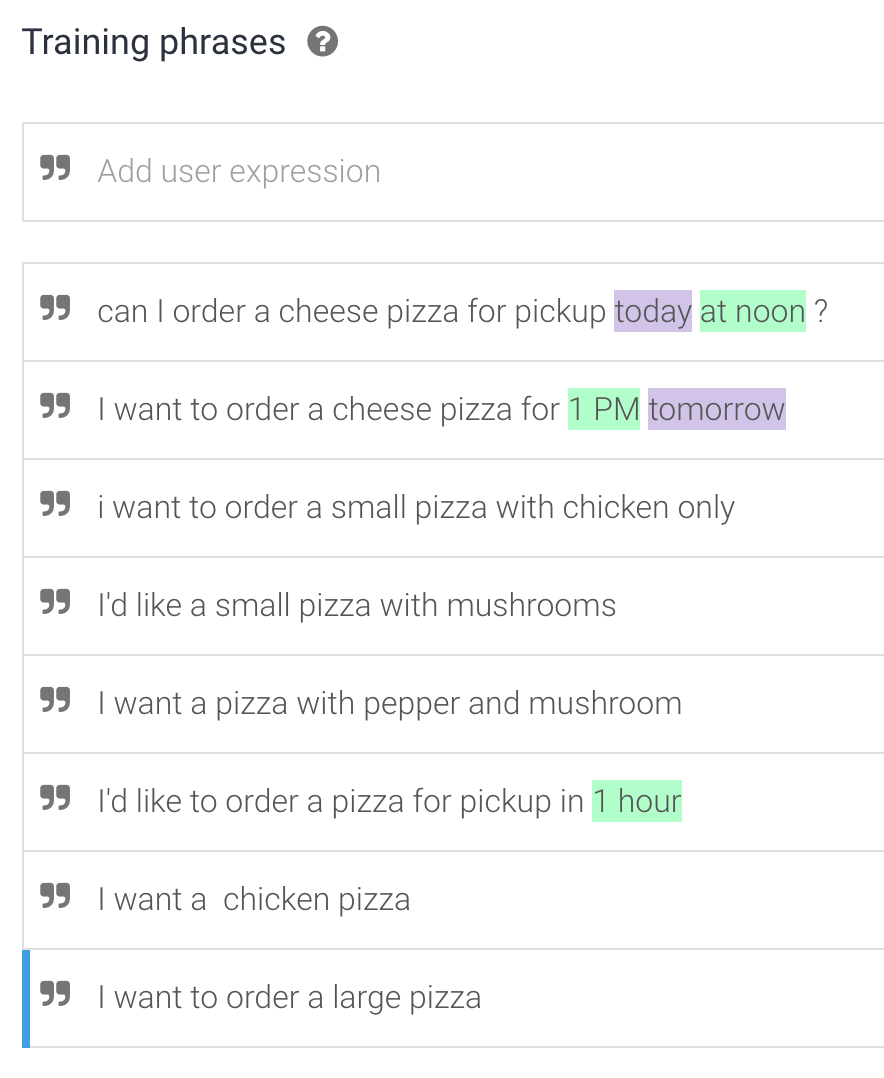This image features an interface with a prominent page displaying a variety of text and elements catered to customizing pizza orders. At the top right, a help icon is visible, suggesting assistance is available. Below, there are multiple fields and examples of user expressions for ordering pizza, including:

- "Can I order a cheese pizza for pickup today at noon?"
- "I want to order a cheese pizza for 1pm tomorrow."
- "I want to order a small pizza with chicken only."
- "I would like a small pizza with mushrooms."
- "I want a pizza with pepper and mushroom."
- "I would like to order a pizza for pickup in one hour."
- "I want a chicken pizza."
- "I want to order a large pizza."

The text is displayed in varying colors including purple, green, and black, providing clear contrasts and categorization for different types of information. The overall layout is designed to facilitate ease of use for placing specific and timely pizza orders.